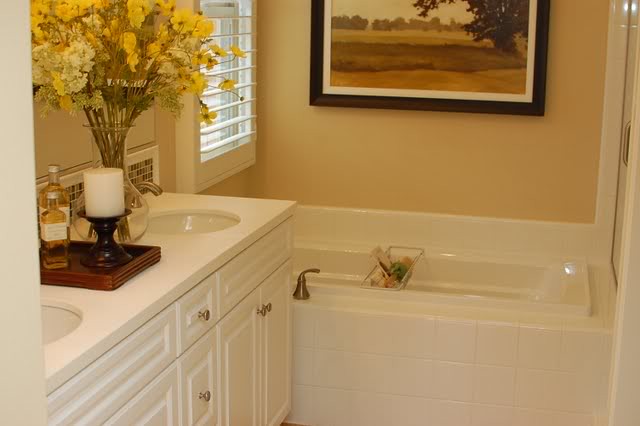This photograph portrays a meticulously clean and aesthetically pleasing bathroom predominantly featuring hues of white, yellow, and various shades of brown. The walls are painted a soothing tan color, giving the room a warm and inviting feel. Above the pristine white ceramic bathtub, a dark brown wooden frame holds a painting that beautifully depicts a lush yellow and green field with scattered trees, adding a touch of nature to the setting. 

A window with a white border and a matching white shade allows for controlled natural light. The bathtub area is further accentuated by a white tile finish, maintaining a consistent and clean design. A sleek metal caddy spans across the bathtub, neatly holding loofahs and an assortment of cleaning items.

Enhancing the bathroom's functionality, a white cabinet is mounted on the left-hand wall, featuring multiple drawers and doors with silver metal knobs for effortless storage. A double sink setup boasts ceramic white basins set into a smooth white countertop. 

Adding to the decorative charm, a brown wooden tray is placed on the countertop, holding a stylish pillar candle holder with a white candle, as well as two elegant glass containers of yellow liquid, likely bath oils. The bathroom is finally adorned with a clear glass vase filled with vibrant yellow and white flowers, bringing a refreshing splash of color to the space.